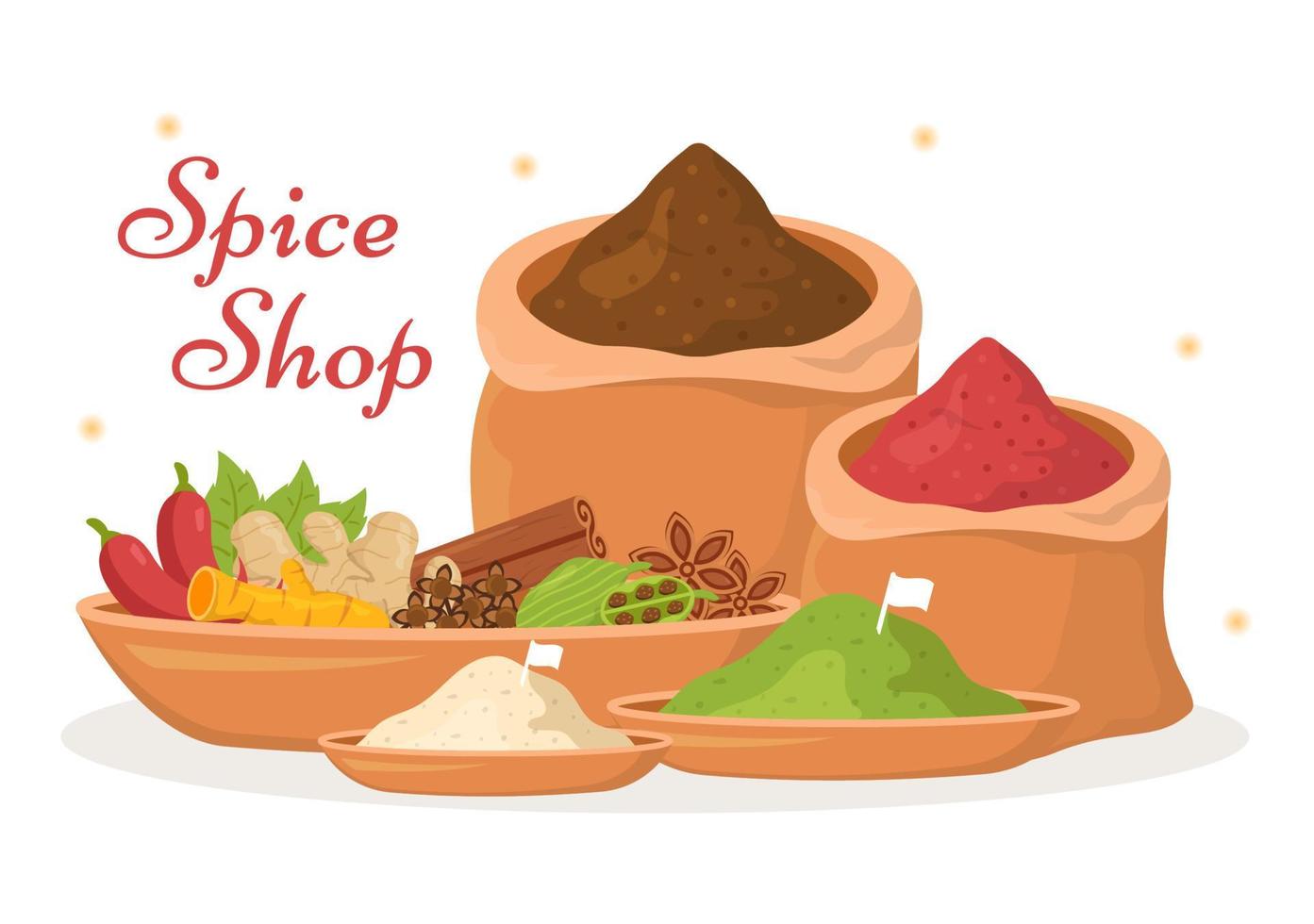In this whimsical, animated cartoon-style image of a spice shop, the background is a clean white with a scattering of blurred yellow and red dots. The top left corner displays the words "Spice Shop" in fancy red cursive text, flanked by tiny gold stars. Centered around an arrangement of various spices, there are five distinct containers: two burlap bags in the background and three terracotta bowls in the forefront.

The largest burlap bag on the left overflows with a brown powdered spice, while a smaller bag to the right is filled with a reddish spice, heaped to a point. In front of these bags, a large, oblong terracotta bowl holds a vibrant assortment of spices including red and yellow peppers, green leaves, ginger root, and neatly stacked cinnamon sticks.

Closer to the viewer, there are two smaller terracotta bowls. The leftmost bowl contains a white, sandy spice with a white flag planted in it, and the slightly larger bowl to its right features a green mound of spice, also with a white flag. The entire scene is supported by a subtle gray circular shadow beneath the containers, lending depth to the charming display.